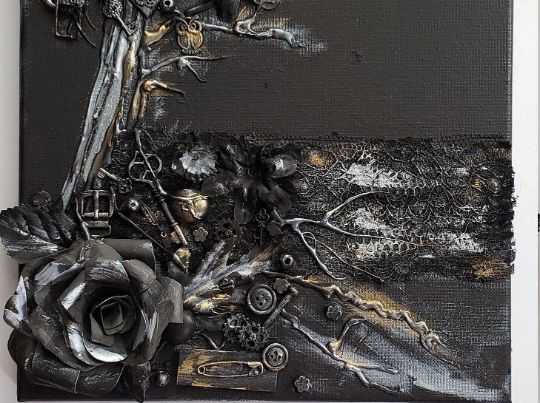The image showcases a detailed close-up photograph of an intricate piece of artwork resembling a book cover, ingeniously assembled with various metallic objects. Dominating the left side is a striking metallic black tree with a few branches, one of which cradles a small owl, finely detailed in yellowish and grey hues. The tree exhibits accents of bronze and gold, lending it a unique metallic sheen. Dangling from a branch is a key, and further down, a watch band clasp is embedded in the artwork. Below these elements, a large black rose crafted from thin metallic sheets rests, its metal leaf adding to the industrial aesthetic. Placed near the rose is a clothespin, a safety pin, and a shirt button, all contributing to the eclectic composition. The bottom half of this artwork is densely populated with these metallic objects, contrasting with the cleaner upper half. The overall color scheme is dominated by shades of grey, bronze, and black, with subtle influences of gold, creating a monochromatic yet artistically rich scene. The piece is bordered by a white frame, which sits on a white surface, accentuating the intricate details and the metallic allure of the objects within the artwork.